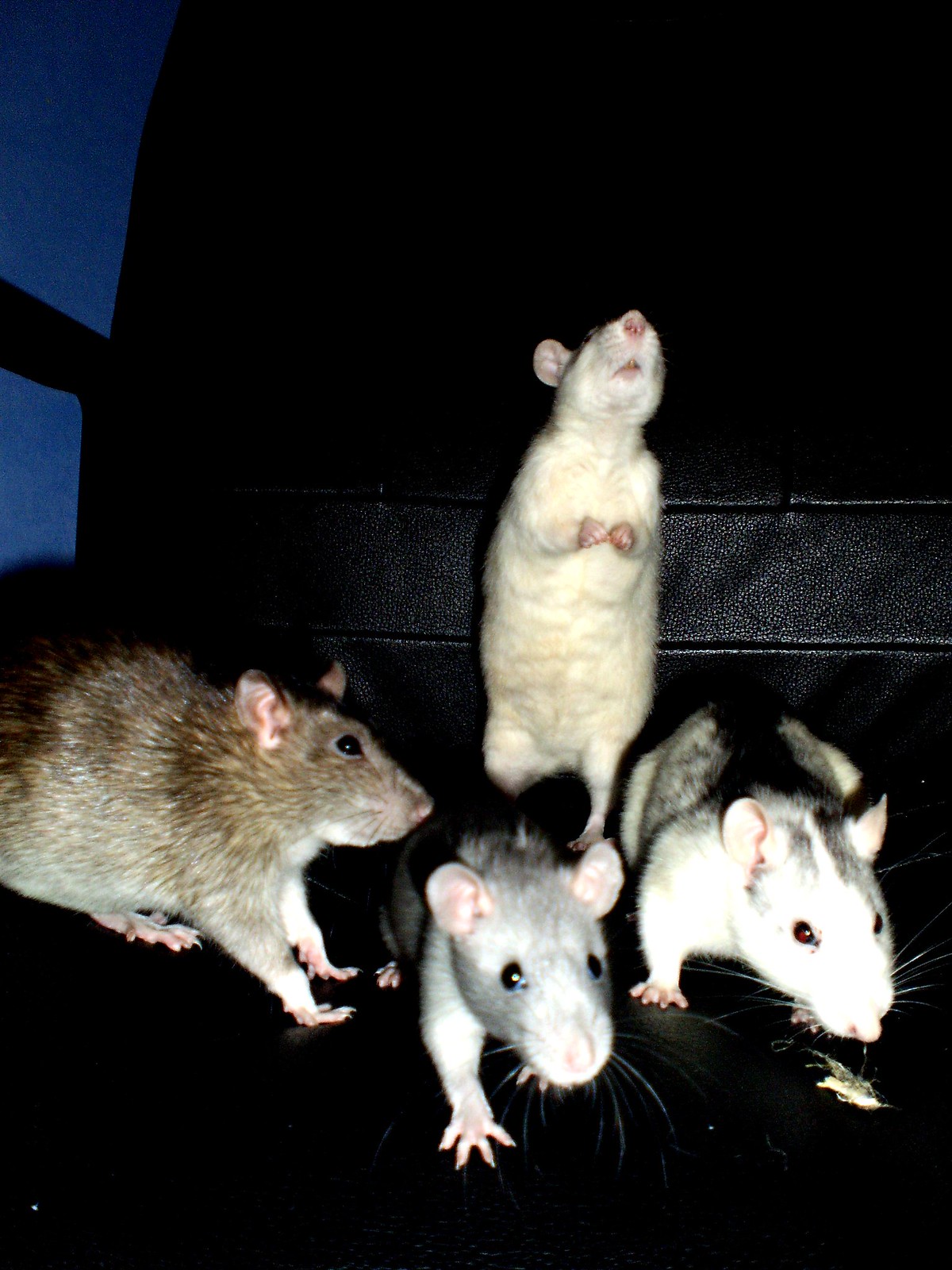The photograph captures four distinct mice perched on a piece of black furniture, which appears to be either an office chair or carrying case, silhouetted against a deep, twilight blue background that suggests the image was taken late in the evening. The furniture features a curving, arch-like design with visible armrests and a strip of black leather across the back. In the foreground, three mice are on all fours: the one on the left has brown fur with white patches, and pink ears, nose, and black eyes; the middle mouse has a gray and white coloration with pink ears, nose, and black eyes; and the mouse on the right is primarily white with gray and black patches, also featuring pink ears and nose, but its eyes appear slightly red due to the camera flash. In the background, the fourth mouse stands on its hind legs, reaching its front paws towards the camera. This upright mouse has a cream-colored underside, and although its head is slightly tilted upward, partially hiding its eyes, its pink nose and ears are clearly visible. Each detail of the scene emphasizes the unique characteristics and variations in color among the mice, as well as the setting they inhabit.